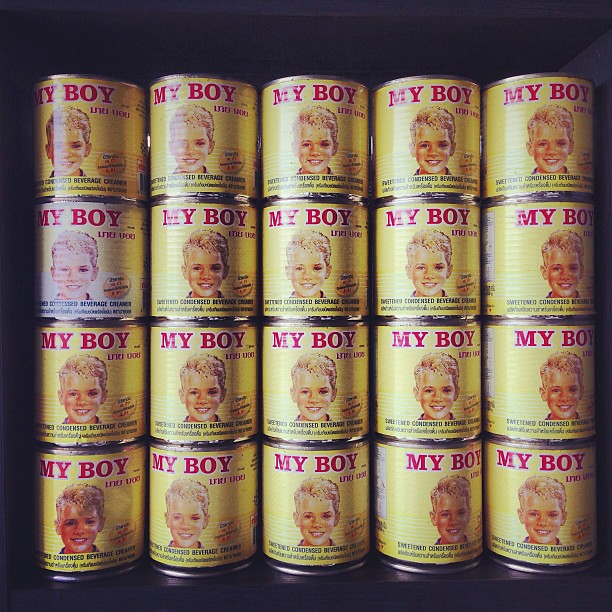This photograph features a neatly stacked pyramid of 20 small, cylindrical cans, reminiscent of the size used for canned Vienna sausages. Each can predominantly features a yellow label with bold red text reading "My Space Boy" accompanied by a smiling image of a young, blonde-haired child on the front. The cans are arranged in such a way that they appear to be almost perfectly identical, except for one near the top left corner which is noticeably faded, giving it a whitish tint. Another can located at the bottom left stands out with a slightly redder appearance on the child's face. The background of the image is pitch black, providing a stark contrast to the bright cans, making them pop visually. The lids and bottoms of the cans are silver, adding a metallic gleam to the overall composition. Although there is some additional text below the image on the label, it is too small to be legible from this vantage point. The image evokes curiosity about the nature of the canned contents, which might be baby food or a similar product.